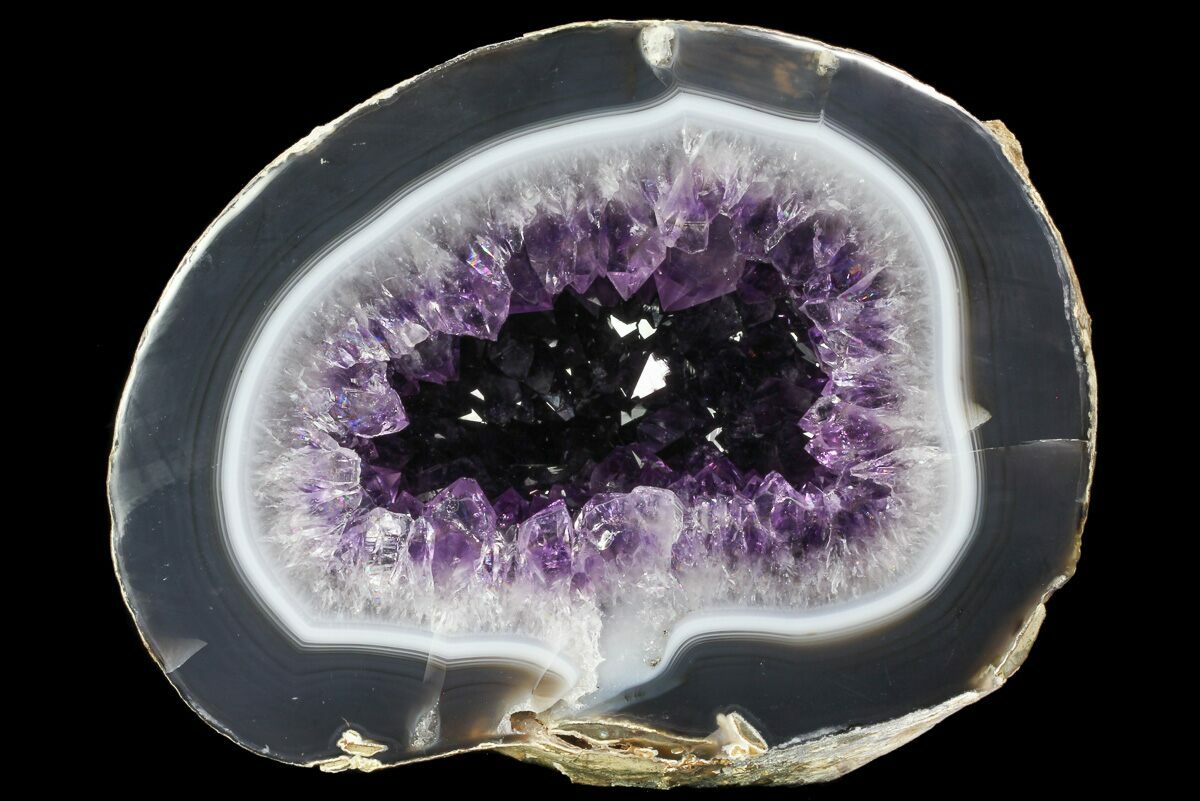This detailed photo showcases a meticulously halved geode against a black backdrop, likely velvet, enhancing its intricate details. The geode itself is almost egg-shaped and large, nearly filling the frame. The outermost band is nearly black, a deep dark gray or brown, giving way to a strikingly thick, creamy, translucent layer, reminiscent of looking into the depths of a dark lake. This milky band transitions smoothly into a thinner, pure white ring that encircles the crystalline center. Inside this white border, jagged crystal fragments emerge, clear at their base and intensifying into vibrant purples as they extend inward, possibly suggesting an amethyst composition. Intricately bound within these layers, these crystals form a mesmerizing, almost icy landscape, with the centerpiece reflecting a stunning amalgamation of clear and purple facets. The contrast between the opaque outer layers and the sparkling inner crystals creates a captivating visual depth.